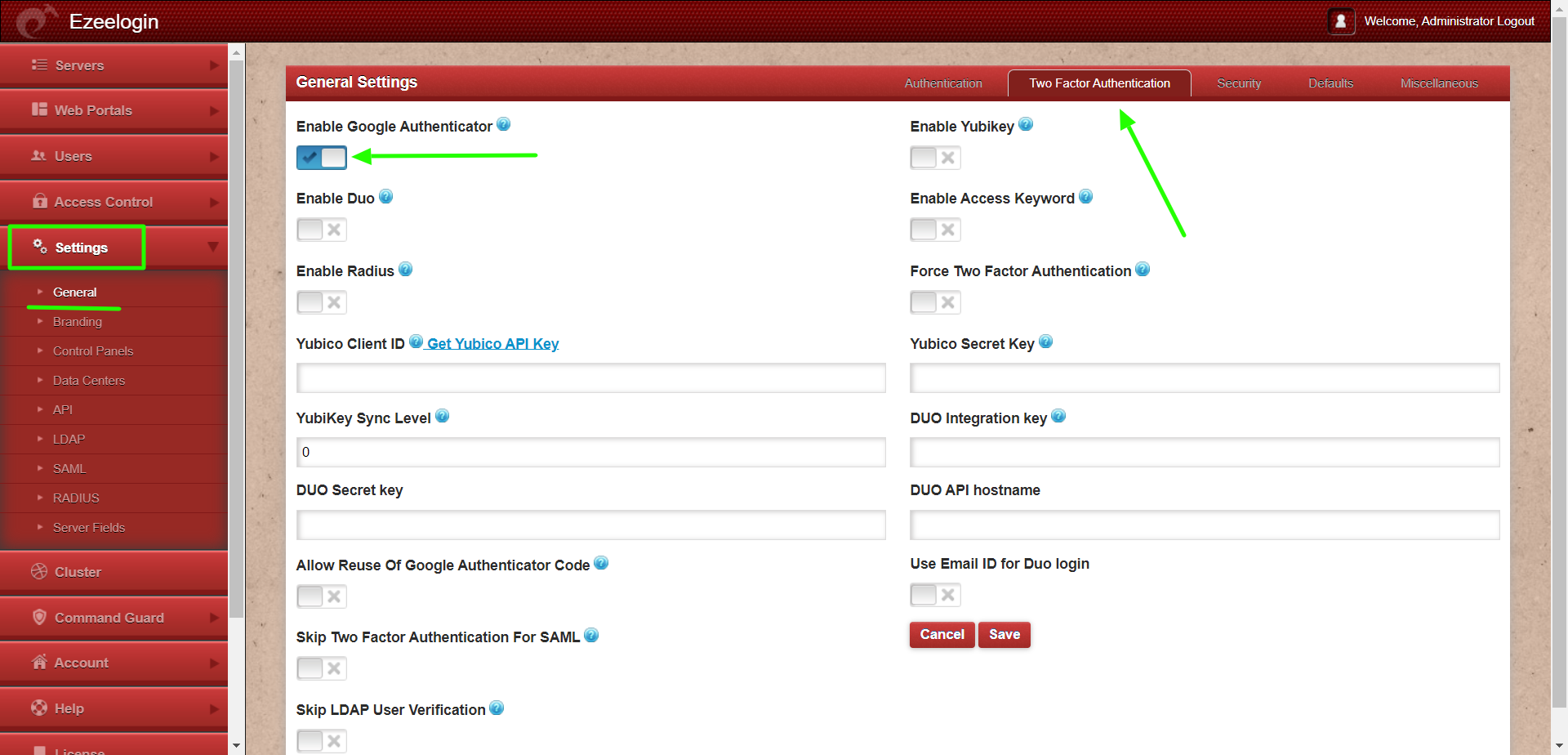The image shows the interface of a platform named "EZ Login," with this title displayed prominently in the top left corner. To the immediate left of the "EZ Login" text is a small, indistinct icon, and to the right of it is a small white profile icon accompanied by the text "Welcome." However, the subsequent text is not clearly readable, but the word "Logout" is visible next to it.

Below the "EZ Login" header on the left side, there is a vertical menu with the options "Servers," "Web Portals," "Users," "Access Controls," and "Settings," each enclosed in dark red boxes and marked with right-pointing arrows. Notably, the "Settings" option features a dropdown arrow and is highlighted, outlined in green. Within the "Settings" section, the submenu "General" is indicated, underlined, and currently selected, opening the main tab to display "General Settings" at the top within a black header.

The main content area reveals configurations related to "General Settings." A green left-pointing arrow is highlighted next to the label "Enable Google Authenticator," accompanied by an empty checkbox. Another green arrow points to a "Two-factor authentication" option. Towards the bottom of the page, there are two buttons labeled "Cancel" and "Save."